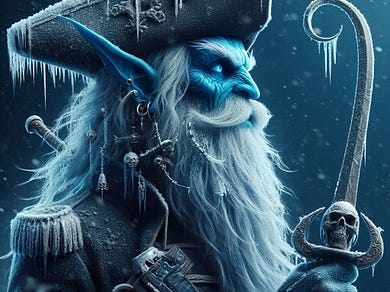This rectangular illustration, approximately three inches wide and two inches high, features a detailed depiction of a ghostly pirate-like creature that appears elf-like in nature. The creature, facing towards the right, has an aged, weathered look with wrinkled blue skin and sharp, elongated ears adorned with multiple pieces of jewelry, including earrings resembling small, skull-shaped bells. His facial features include a long, downwards-pointing nose, thick white eyebrows, blue eyes, and a long white beard and mustache. He's clad in a captain’s uniform with icy embellishments, including a dark tricorn hat, from which icicles dangle. His coat, reminiscent of a general's, features gold designs and threads hanging decoratively from the shoulder. Gripped in his right hand is a distinctive silver sword with a left-curving tip and icicles forming along the curved portion. The hilt of the sword, adorned with a skull motif, curves on both sides. The entire scene is rendered in various hues of blue, reinforcing the frosty, ghostly atmosphere. The image is cut off just below the shoulders, hinting at the figure’s ominous presence and authority.